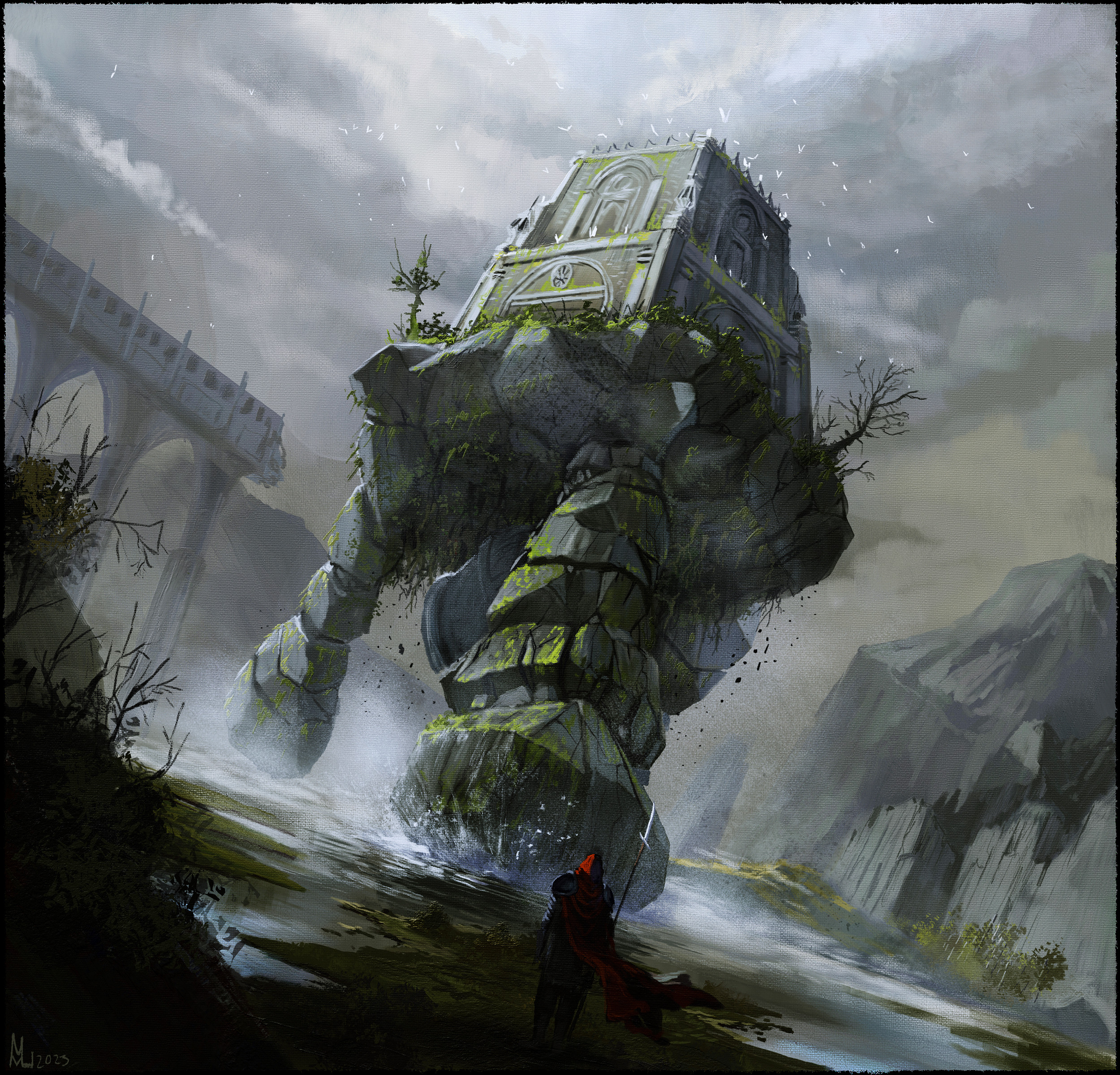**Detailed Caption:**

This square, color illustration epitomizes the fantasy genre, capturing an awe-inspiring scene of a tall, ancient city or castle perched atop a massive, textured megalith rock that juts dramatically out of a turbulent, angry ocean. The predominant hues of gray, black, and light green convey a somber, mystical atmosphere. A small, solitary figure stands in the foreground, gazing up in wonder at the colossal rock formation and the majestic structure upon it. Adding to the ethereal quality, white birds soar towards the castle, further enhancing the sense of mystery and grandeur. The churning waters below are shrouded in fog with highlighted sprays, while the interplay of light and shadow across the entire image contributes to its depth and texture. This illustration, while retaining the meticulous detail of pen and ink strokes that move in various directions to create rich textures, appears to be a digital artwork, blending traditional and modern artistic techniques to create a captivating visual narrative.